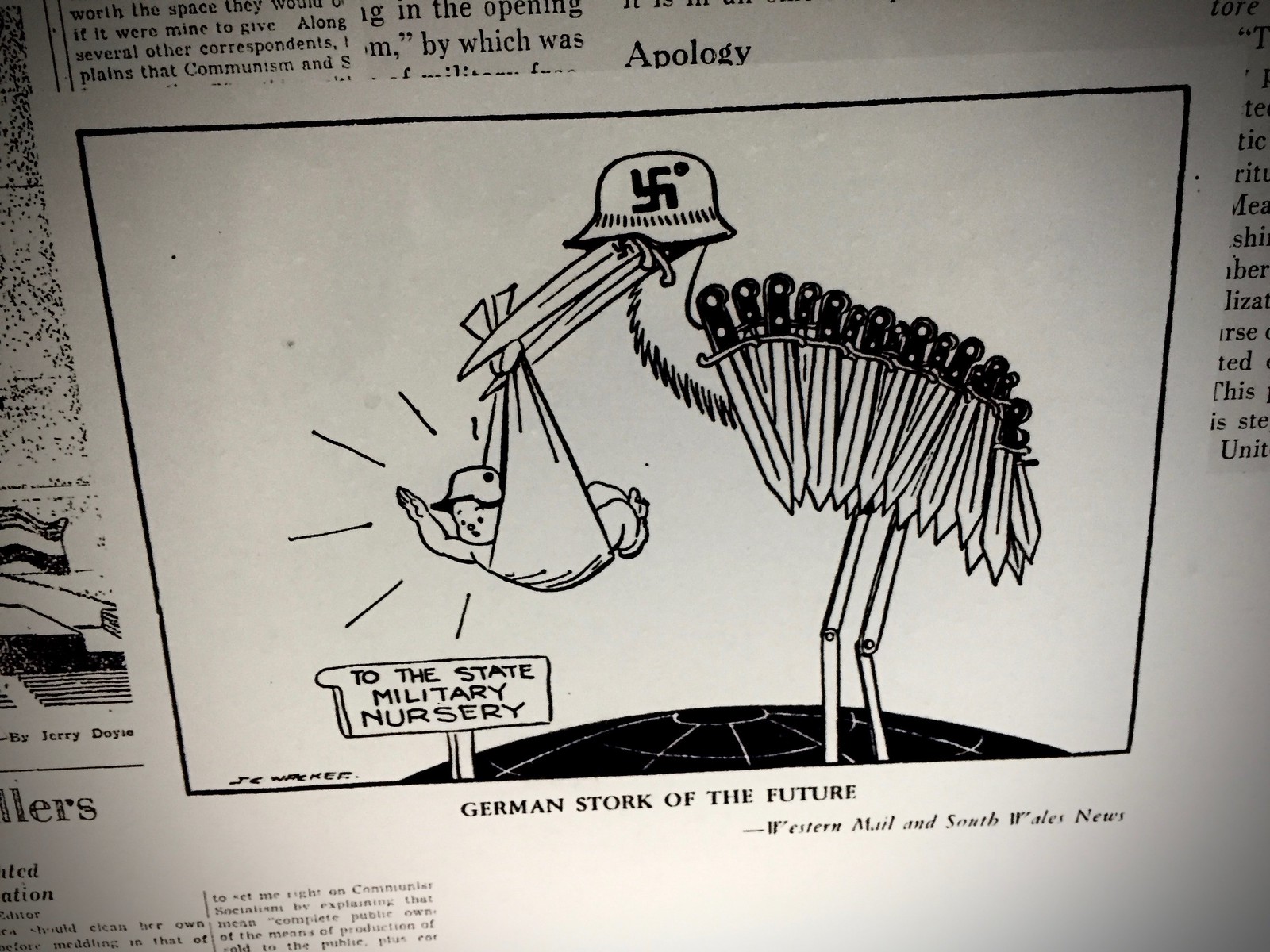This black-and-white political cartoon, seemingly extracted from an old newspaper, portrays a "German Stork of the Future" and prominently features stark World War II imagery. At the center, a stork with a grotesque twist is depicted: it dons a Nazi helmet emblazoned with a swastika, and its body bristles with an array of knives and bayonets. The stork clutches a bundled baby in its beak, itself adorned with a German helmet, suggesting a militaristic future. They stand upon a globe, underscoring a worldwide menace. A sign to the left reads, "To the State Military Nursery," alluding to the regimented fate awaiting future generations. This chilling illustration is labeled at the bottom with the caption, "German Stork of the Future," along with a note, "Slash Western Mail and South Wales News," indicating its publication source.